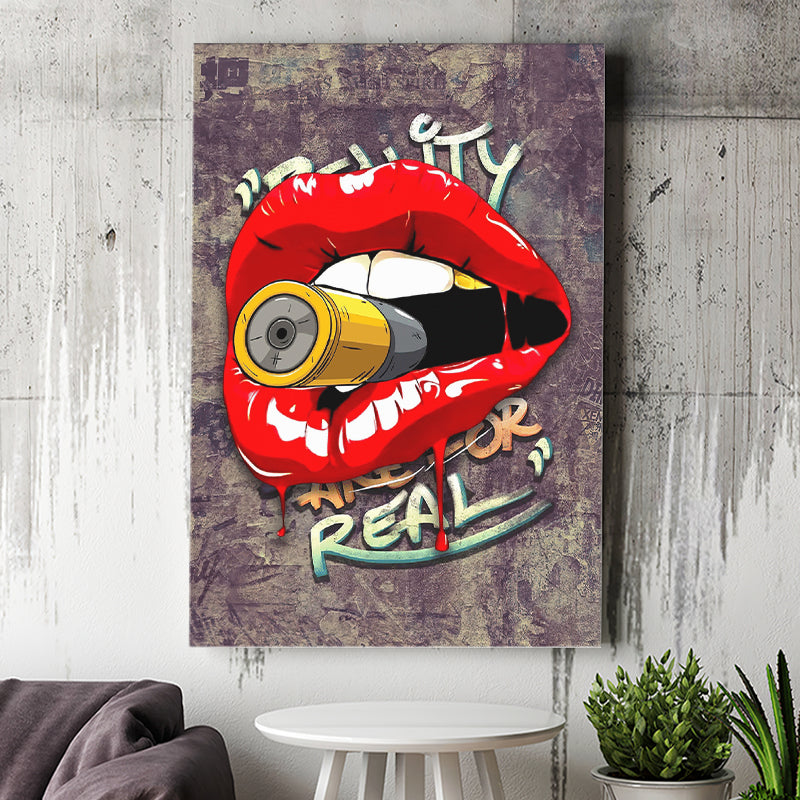The image is a detailed color photograph featuring a prominent piece of pop art with a gritty, urban aesthetic. Displayed centrally on a textured purple and beige wall, the art is portrait-oriented and vividly depicts a striking set of red lips parted to reveal white teeth, with one of the front teeth adorned with a distinctive gold crown. The lips are gripping a gold-tipped bullet, which adds an edgy intensity to the artwork. Notably, the bullet's casing is gold, transitioning to a gray tip, while the lips appear to be dripping in red, resembling blood. The backdrop includes partial graffiti tagging that complements the urban theme.

Beneath this compelling art piece, we see a white circular table with five or six legs, providing a minimalist, modern contrast. To the left of the table, there's a glimpse of a black couch, showing just the top parts of the seats. To the right, two potted plants add a touch of greenery: the nearer plant has numerous small green leaves reminiscent of Brussels sprouts, and the other features long, bladed leaves with little spikes, akin to cactus leaves. The entire scene is captured in a square format, with the arrangement of elements emphasizing the art's raw, provocative impact within a realistic representational style. The word "REAL" is spelled out at the bottom of the art, anchoring its bold message.